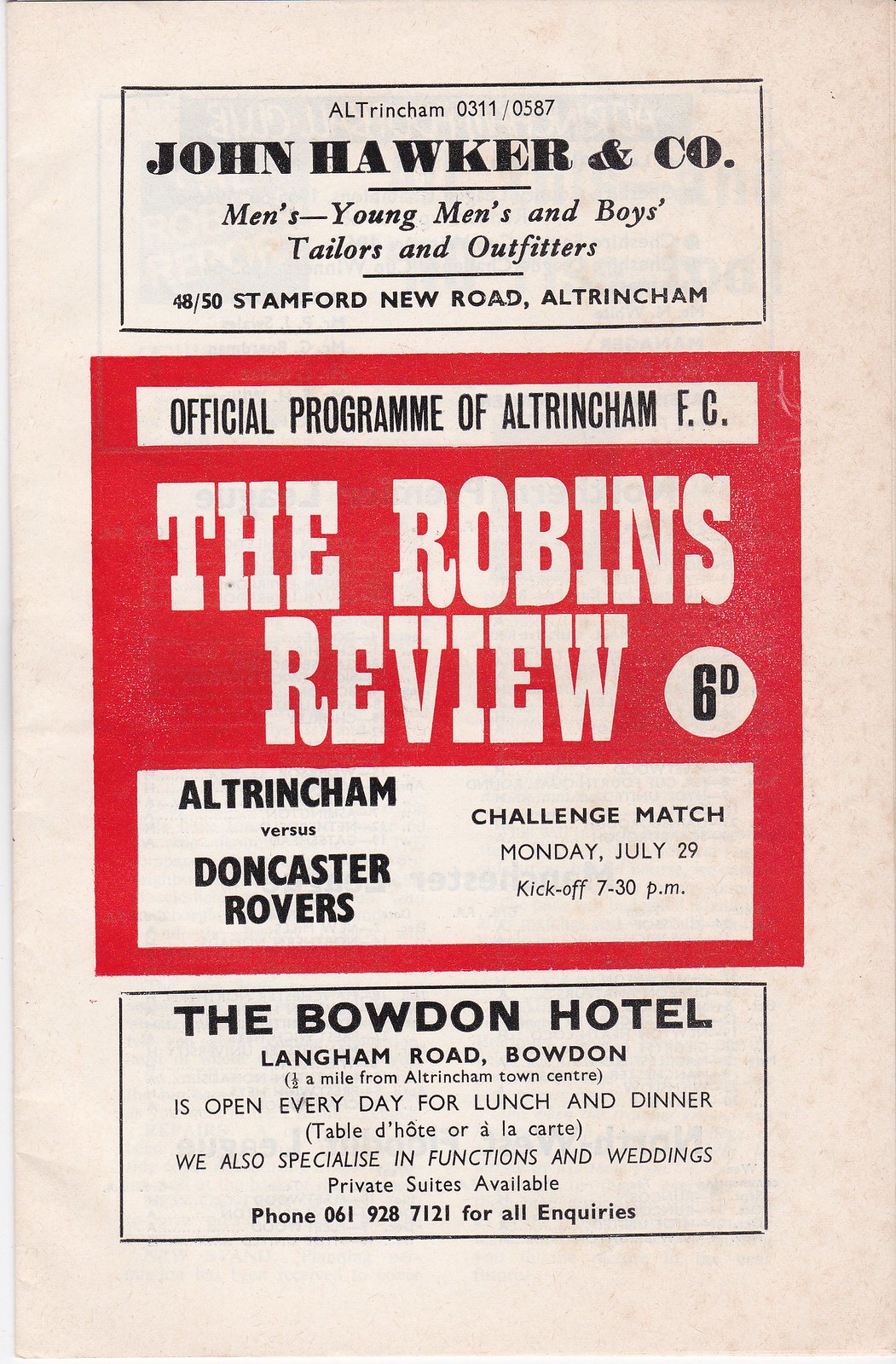This is a photo or scan of an old sports program cover, likely from the 1960s, featuring a blend of off-white, red, and black colors. The cover has three distinct sections, separated by black rectangular borders. The top section displays an advertisement for John Hawker and Company, located at 48/50 Stamford New Road, Altrincham, describing themselves as "men's, young men's, and boys' tailors and outfitters." Just below this, in the same top section, it states in black text, "Official program of Altrincham FC." The middle section is dominated by a red background with white bold text proclaiming "The Robins Review" and the match details: "Altrincham versus Doncaster Rovers, Challenge Match, Monday, July 29, kickoff 7.30 p.m." Additionally, "6d" is mentioned off to the side, reflecting the cost or issue number. The bottom section features an advertisement for the Bowdon Hotel on Langham Road, Bowdon, which announces it is open daily for lunch and dinner and specializes in functions and weddings, providing a phone number for all inquiries. This cover not only highlights the sporting event but also includes prominent sponsor advertisements.